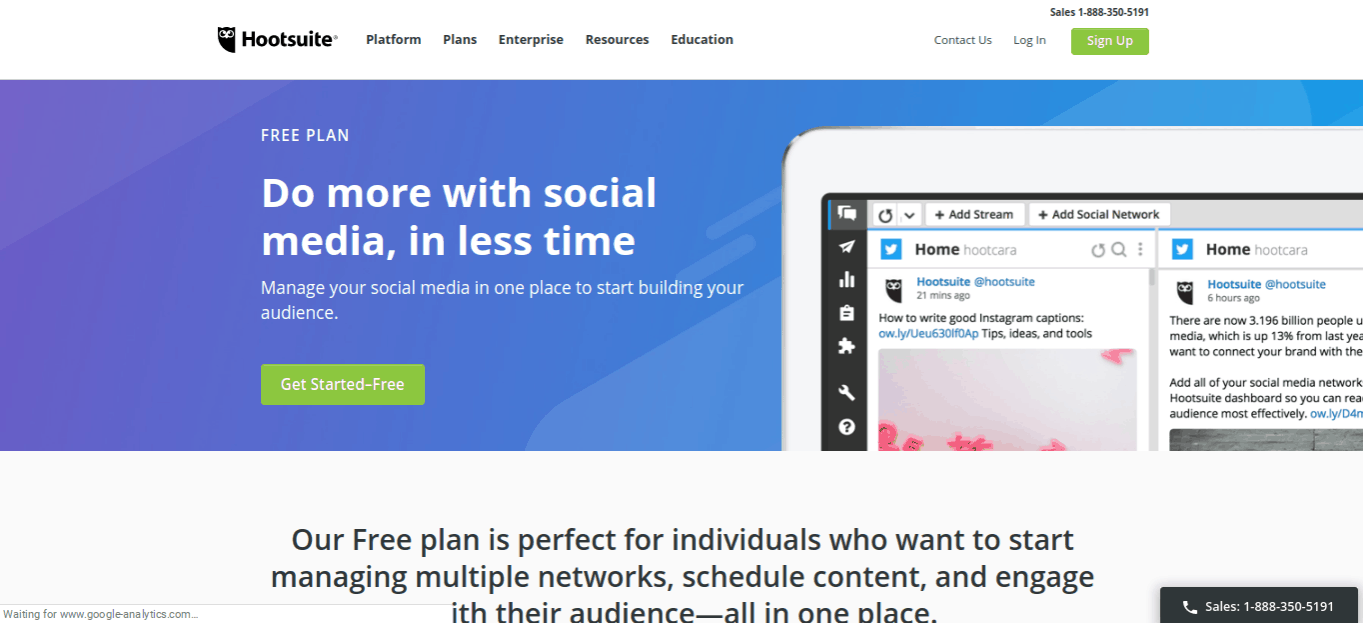The image is a cropped screenshot of the Hootsuite homepage, characterized by a clean, white background. At the top left of the page is the Hootsuite logo in bold black font. To the right of the logo, five navigational categories are listed in small black font: Platform, Plans, Enterprise, Resources, and Education. Just past these categories, in very small blue font, are the options "Contact Us" and "Log In." To the right of these, a small, green rectangular "Sign Up" button is prominently displayed, featuring the words "Sign Up" in white at its center. Directly above this button is a sales telephone number, presumably for customer inquiries.

Beneath the top navigation bar, there is a very long rectangular header with a striking purple background. The header begins with "Free Plan" at the top in small letters. Directly below, in large, bold white letters, it reads, "Do More with Social Media in Less Time." Beneath this compelling tagline, in smaller white letters, it further explains, "Manage Your Social Media in One Place to Start Building Your Audience." Towards the bottom of the header, a green rectangular bar with the call-to-action "Get Started Free" appears in white letters.

To the right side of the header, there is a partial view of the top-left edge of an iPad screen displaying Twitter posts tweeted by Hootsuite. The partial iPad image and the combination of text and visuals reinforce Hootsuite’s focus on social media management and engagement.